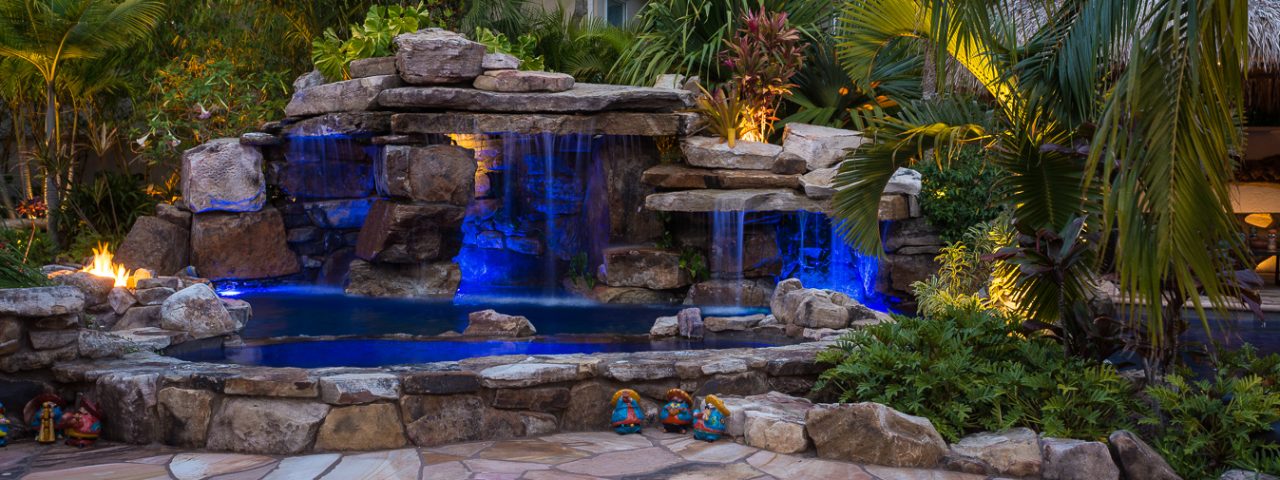This wide landscape photograph captures a serene garden oasis, centered around a manmade waterfall feature and a naturalistic swimming pool, glowing neon blue under the night sky. The foreground showcases a stone pathway, inviting visitors to walk or sit on flat-topped rocks amidst small decorative elements. At the heart of the scene is a meticulously crafted waterfall, where cut square stones are artfully stacked, and water is piped over them, enhanced by blue LED lights. This focal point is flanked by a lush array of tropical greenery, including palm fronds and ferns, adding to its paradise-like ambiance. A fire pit flames on the left, while three small statues can be seen on either side of the pool. Behind the waterfall, the rock structure mimics a cave, creating an intimate grotto effect against the pool's calming midnight blue hue, amplified by additional lighting. The overall effect is one of luxurious tranquility, devoid of people or text, but rich in natural beauty and sophisticated design.